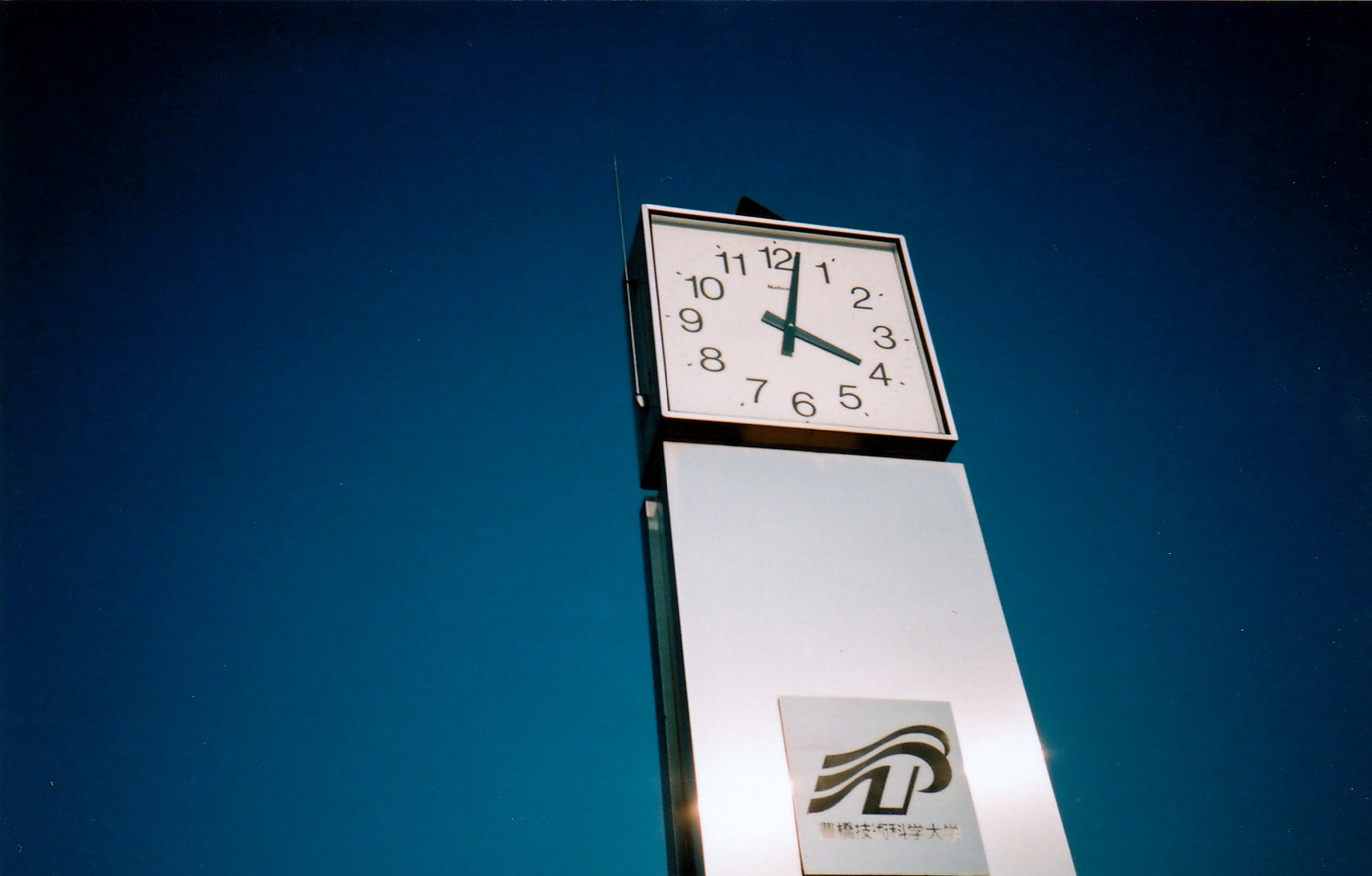The image features a prominently displayed outdoor advertising or business sign, which is likely the entrance sign of a mall or a similar establishment. This vertical structure is crowned by a large square clock, with a striking white face and bold black numerals. The clock displays the time as two minutes past four, with easily visible large minute and hour hands. Adjacent to the left side of the clock, there is what looks like an antenna or flagpole, adding an additional element of height to the sign.

The photograph is taken from a low angle, positioned below and to the left of the clock, emphasizing the structure’s towering presence against a dark, cloudless blue sky. Below the clock, the rectangular section of the sign appears to be made from a polished metal, likely aluminum, reflecting a sleek, modern aesthetic. Atop this metallic segment is a smaller rectangle or square sign bearing a flag-like 'T' symbol accompanied by oriental script beneath it. The clear details of the clock and the precise symbols lend a professional and well-maintained impression to the establishment it represents.